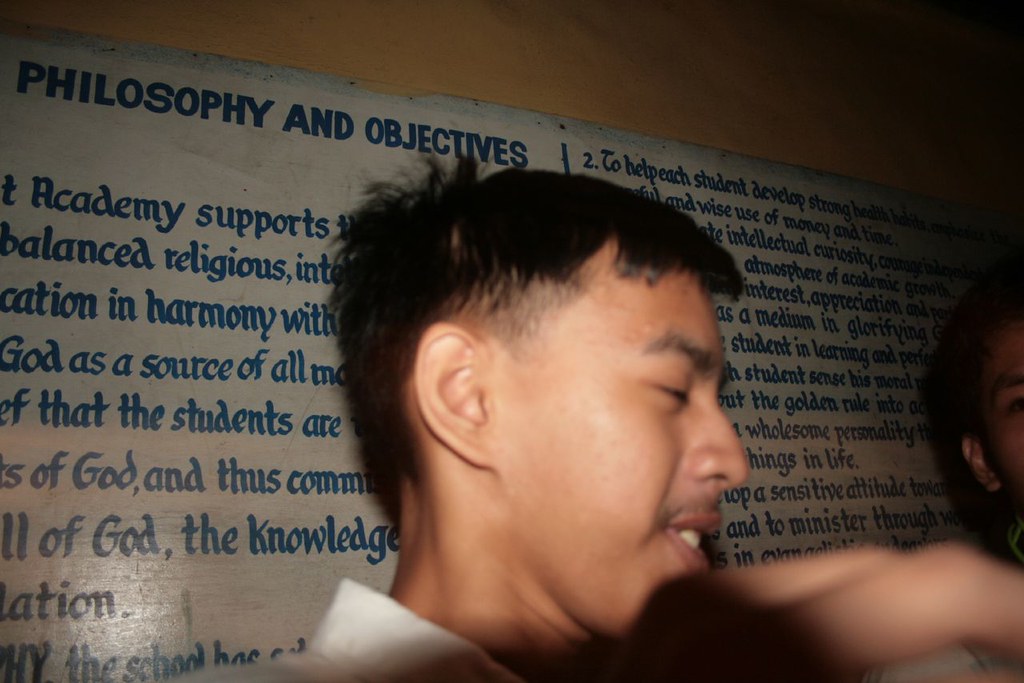The photograph captures a young man, likely in his 20s or 30s, who appears to be of Asian or possibly Mexican descent, standing in a dimly lit room. The lighting primarily from the camera illuminates his short, very dark, straight hair which is slightly unruly with a fade at the sides. He has a slight mustache and bushy eyebrows, his eyes nearly closed, giving an impression of discomfort or shyness. He wears a white collared shirt, and his hand appears close to the camera, hinting at an unposed, candid moment. Behind him, a large orange board with blue text in varying degrees of clarity spells out "Philosophy and Objectives" and discusses the principles of an academy promoting balanced religious thoughts, harmony with God, and the development of strong beliefs, wise use of money, and time. Just barely visible beside him is the side of another person's face, contributing to the sense of a populated, yet focused setting.